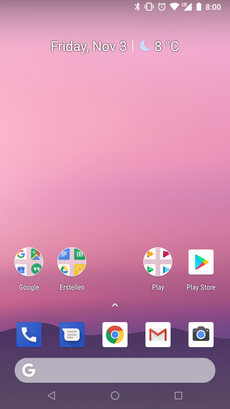This image showcases a smartphone's home screen with various details. At the top of the screen, standard icons indicate the time, battery level, connection status, Wi-Fi, and Bluetooth. The date displayed is Friday, November 3rd, and the weather shows a temperature of 8 degrees Celsius with a half-moon icon, suggesting it's nighttime.

The background is a gradient purple that transitions to a darker purple at the bottom. Dominating the screen are four folders: Google, an unreadable label, Play, and Play Store. These folders likely contain multiple apps within them. 

At the bottom of the screen is a row of five primary icons: Phone, Text, Chrome, Mail, and Photos. Just above this row is a prominent Google search bar. Below the main apps and folders, three additional icons are positioned against the darker portion of the background, for a total of three visual layers.